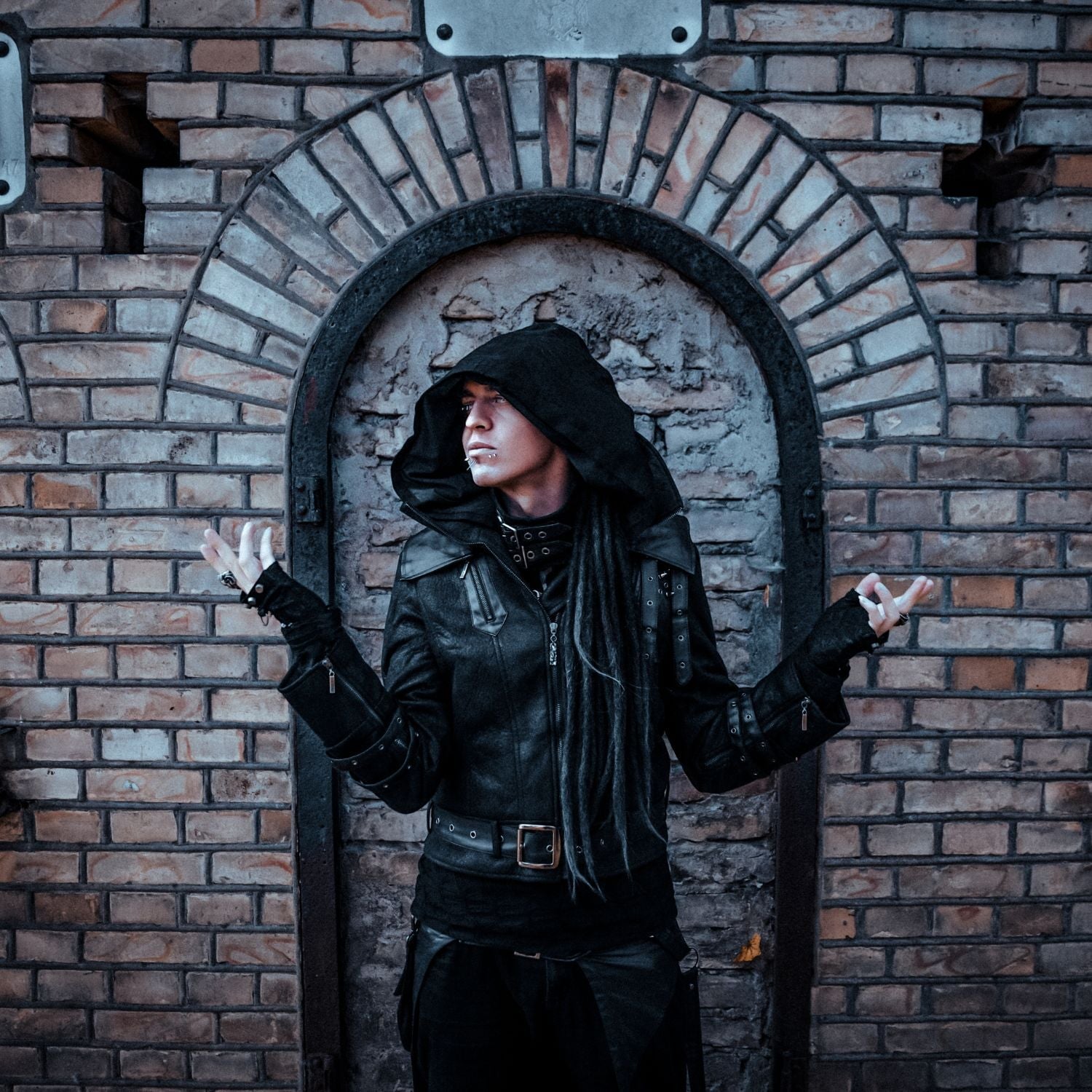A young man, seemingly in his 20s, stands in front of a medieval gothic-inspired brick facade. The intricate stone wall features an arched doorway, sealed off with bricks and adorned with metal trimming and cross symbols on either side. The man, clad in modern black leather attire, including a hooded jacket and pants, exudes a gothic, gangster-like vibe. His long black dreadlocks peek out from under his hood, and his face is strikingly adorned with numerous piercings around his lips, nose, and eyelids. With arms raised and open, he gazes to the left, seemingly in a moment of wonder. The image is dominated by dark tones—black, shades of grey, and brown—reflecting the overall somber and gothic atmosphere.